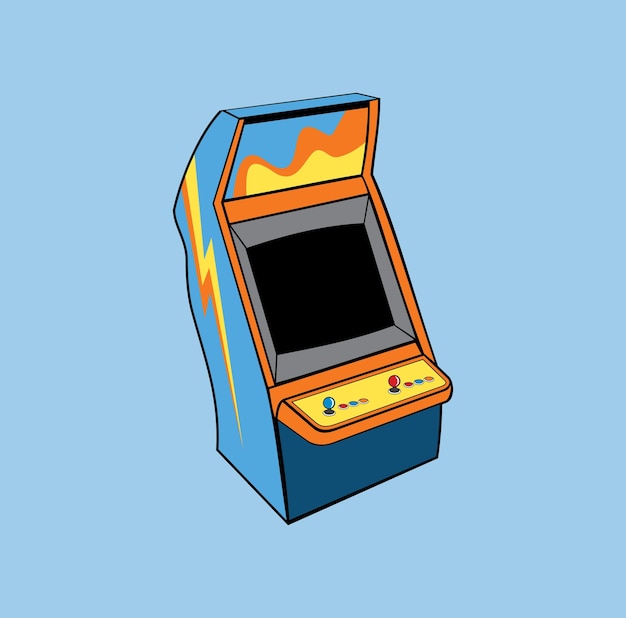The image is a detailed color illustration rendered in a square format, featuring a cartoon-style arcade gaming machine set against a solid light blue background. The machine, which appears to be drawn with light and dark blue tones, is positioned at an angle where the front panel faces the top right and the corner of the machine points towards the bottom center. 

The left side of the arcade machine displays a vivid yellow lightning bolt with an orange shadow effect. On the top, there's a whimsical, swirly pattern in orange and yellow. The monitor at the center front of the machine is framed in gray, with a solid black screen. Below the monitor, the control panel is yellow, featuring two joysticks and an array of buttons. The joystick on the left is light blue, while the joystick on the right is bright red. Each joystick is surrounded by a set of buttons of varying colors, including red, green, and orange. The overall composition suggests a retro gaming aesthetic, highlighted by its bright, contrasting colors and simple yet evocative design elements.